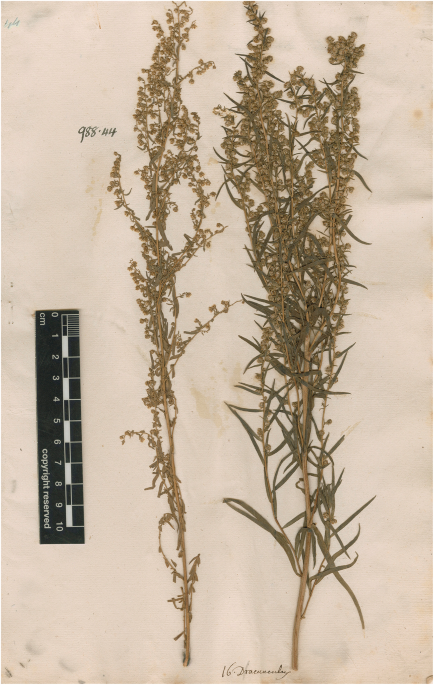The image showcases a vertical, portrait-oriented photograph of two dried plant specimens, laid out side by side on a weathered, pinkish-beige parchment. The parchment appears to be from a previous century, marked with stains and a signature, difficult to decipher, followed by the number '16'. Above the right plant, the notation '988.44' is inscribed, indicating some form of botanical classification. To the right of the parchment runs a vertical black-and-white centimeter scale, ranging from 0 to 10 cm, used to measure the plants' lengths. 

The plant on the left features small, frequent leaves along its stem, primarily consisting of buds. In contrast, the plant on the right exhibits a combination of leaves and buds, with leaves characterized as long and thin, displaying a yellowish-green hue. Both plants share a considerable height and exhibit a dark amber tint, lending an aged artistic quality to the photograph. The overall ambiance suggests an archival botanical illustration with a reserved copyright notice.